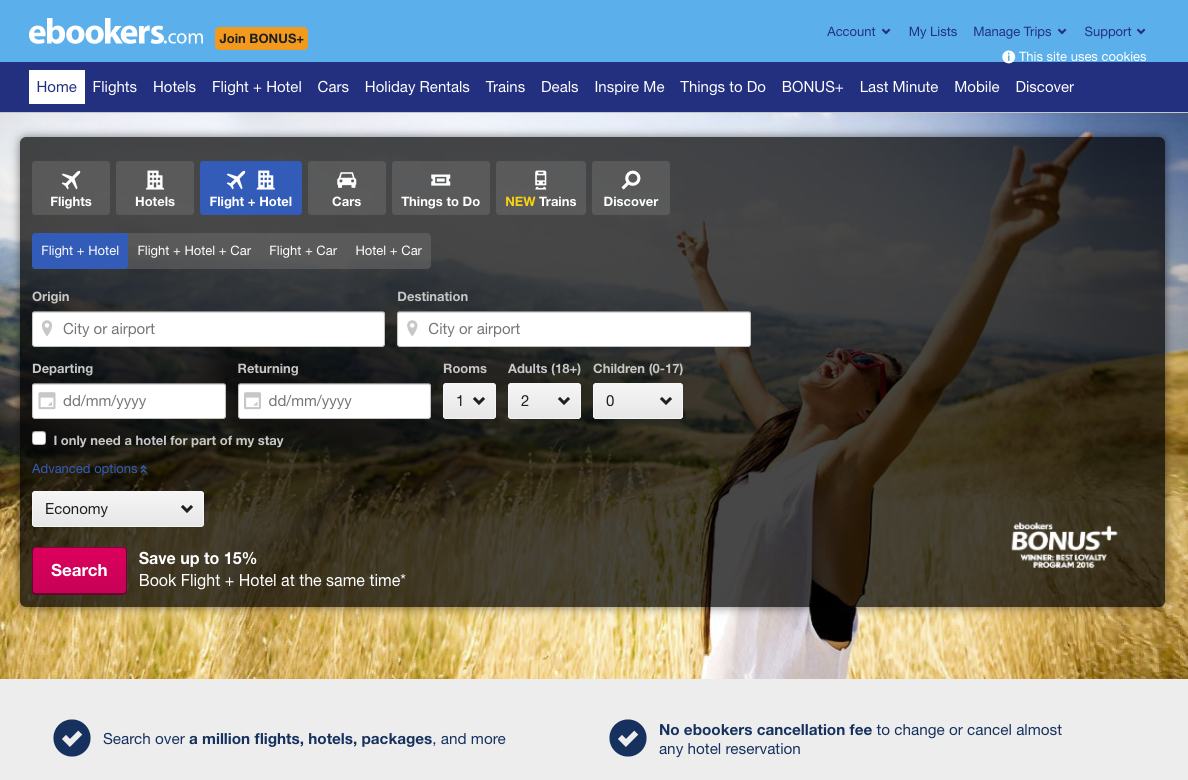This is a detailed screenshot description of the ebookers.com homepage. At the top of the page, there is a light blue banner. In the far left corner of the banner, the text "ebookers.com" is displayed in all lowercase letters with a white font. Next to it, enclosed in a gold rectangle, the text "join BONUS+” is written in black font. On the right-hand side of the banner, there are menu options including "Account," "My List," "Manage Trips," and "Support," each accompanied by a pull-down menu arrow, all written in blue font.

Below this banner, there is a navigation bar that spans the entire width of the page and is colored dark blue. The text within this bar is predominantly white, except for the "Home" button, which is highlighted in white with blue font, indicating that it is the current selection. The other navigation options include "Flights," "Hotels," "Flight + Hotel," "Cars," and more, suggesting that this is a travel website.

The main background image showcases a woman standing in a desert with her hands raised in the air, appearing to celebrate while looking towards the sun. She is wearing sunglasses and a white tank top with the sleeves cut off.

Overlaying the background image, there is a black search input box. This box allows users to enter details about their travel plans, including departure and destination points, and travel dates. Below these input fields is a large, clickable red "Search" button that users can press to get travel results.